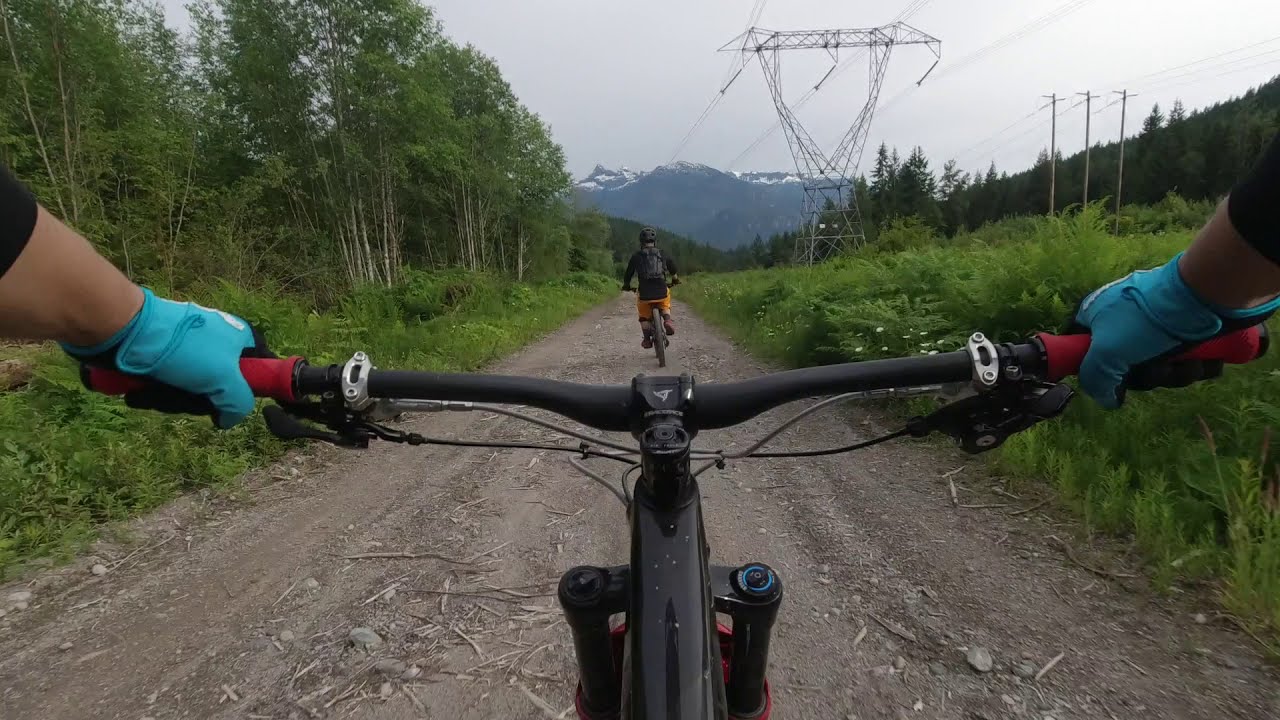This image captures the thrill of two people mountain biking on a scenic dirt trail, taken from the perspective of one of the cyclists. The trail is rugged, scattered with dirt, twigs, and rocks, flanked by grass, bushes, and tall trees with lush green leaves. The rider in front is dressed in a black t-shirt, orange shorts, a black helmet, and a black backpack, and is pedaling a black mountain bike with red handlebars. The trailing cyclist, whose point of view we share, wears bright teal gloves and grips the black and red handlebar of their mountain bike. Overhead, the sky is overcast and gray, adding a moody atmosphere to the setting. In the distance, a majestic mountain capped with snow looms ahead, while on the right, power lines and poles stretch parallel to the trail. The scene is characterized by its natural beauty and the sense of adventure as the two cyclists navigate this vibrant wilderness path.